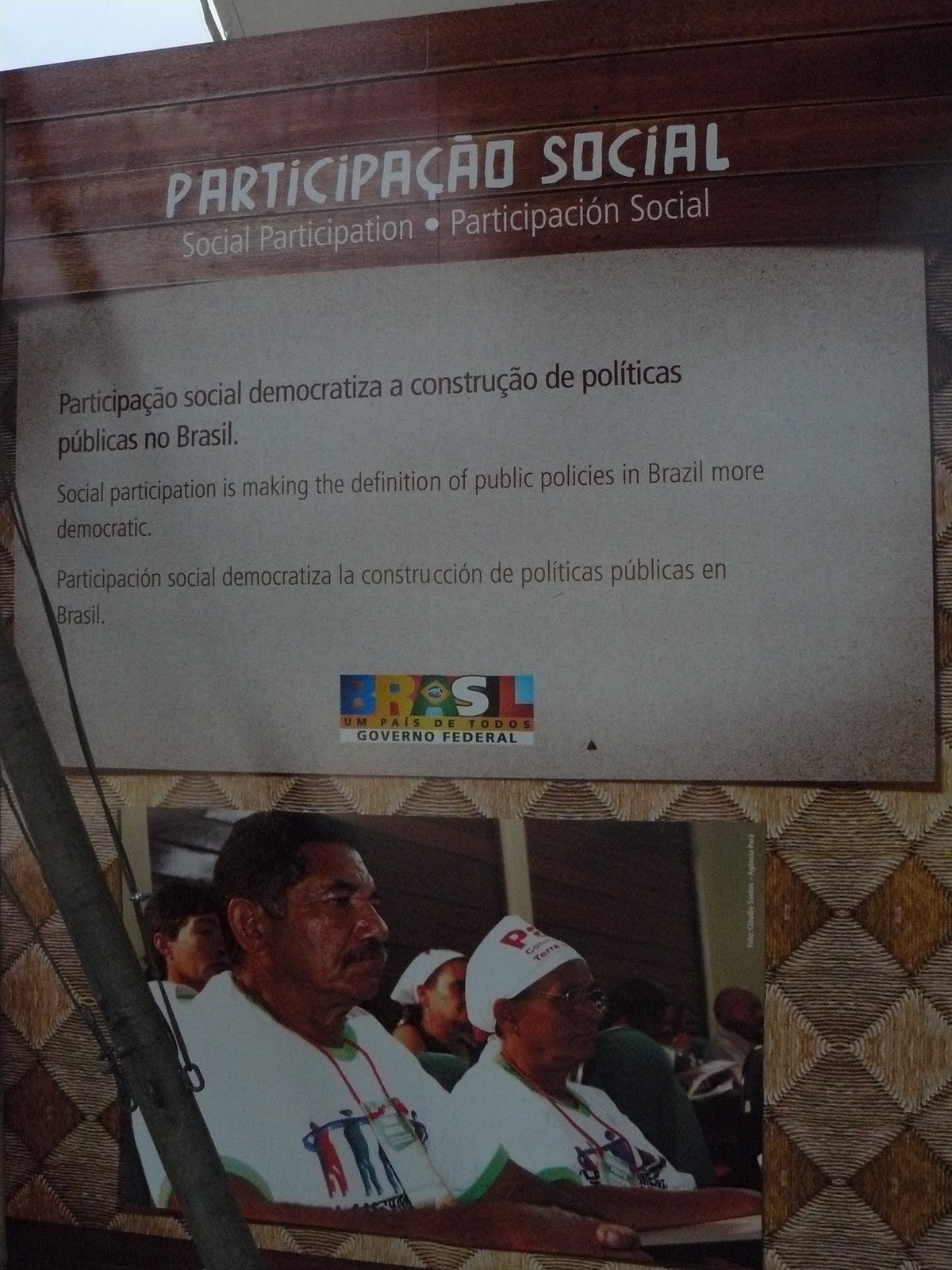The image depicts a slightly aged Brazilian sign, presenting text in both Portuguese and English, against a wall adorned with a distinctive diagonal pattern of brown and beige triangles. The top portion of the sign is framed by wooden planks with "Participação Social" (Social Participation) written in white. Beneath this title, the text elaborates in English: "Social Participation is making the definition of public policies in Brazil more democratic." Further down, a vibrant logo spells out "Brasil," accompanied by the phrase "Um país de todos, Governo Federal." Below this, a photograph captures a slightly elderly couple, seemingly of native Brazilian descent, dressed in matching white t-shirts featuring a design of people standing or holding hands. The woman wears a white cap with red lettering, both individuals looking ahead, suggesting involvement or protest. The sign, set amidst a patterned background, subtly indicates its vintage nature through its subdued and grainy tones.